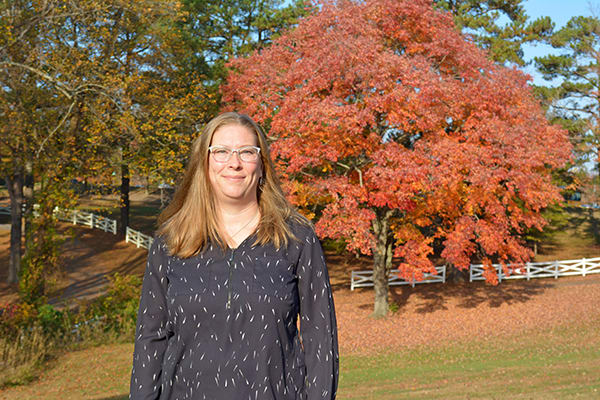In an open grassy field, a white woman stands off to the left of the frame, smiling warmly at the camera. She has light brown, shoulder-length hair and wears clear, white-trimmed glasses. Her black long-sleeved v-neck blouse is sprinkled with white dots resembling raindrops. The photo is a wide vertical shot that captures her from the waist up. In the background, a striking dark red leaf tree stands prominently in the center, surrounded by a mix of green and yellow leafy trees. Under the colorful foliage, a white plank fence stretches horizontally, curving upward on the left. The ground is a mosaic of green grass and patches of brown sand. The blue sky peeks through the branches of the trees, indicating it's daytime and likely fall, given the vibrant leaf colors. The scene exudes a natural, serene outdoor atmosphere, with no text or words in the picture.